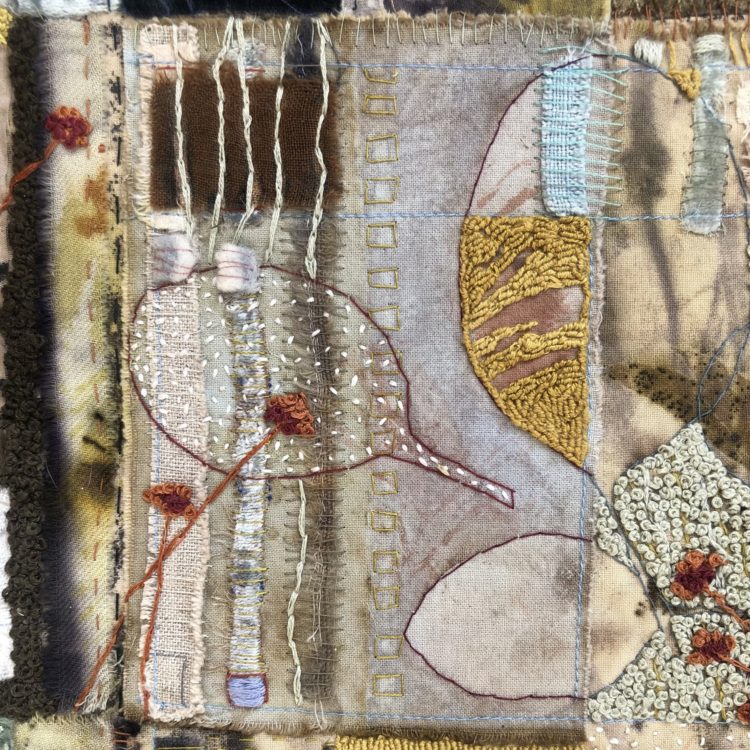The image showcases a detailed close-up of a textile piece, likely an antique or vintage handcrafted item. The fabric, which is possibly a linen or quilt-like material, features an intricate mix of hand-stitched details in an array of colors including white, red, black, yellow, blue, and brown. The craftsmanship includes elements of embroidery and crocheted chain work, integrating various textured fabrics that give it a raised, tactile quality. Prominent features include flowers situated at the bottom left and right corners, which are accented with reddish stems. The patterns are eclectic, with some stitchings resembling outlines of leaves or tennis rackets. The overall design, potentially reflecting Native American or other cultural influences, evokes a sense of historical and artistic significance, despite its somewhat inconsistent motifs.